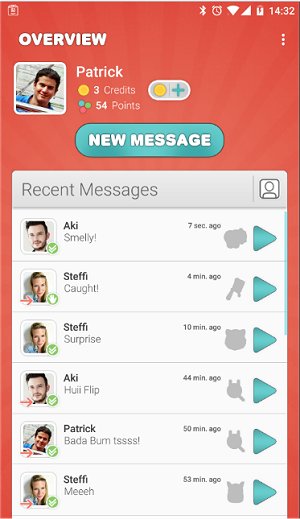The image features an orange background with several notable icons and text elements distributed across it. On the left side, an unidentified icon is visible, adjacent to which a series of recognizable icons are lined up horizontally. These include the Bluetooth, alarm clock, and fan icons, followed by a right-angle triangle in white, a mostly full battery icon, and the time displayed as 14:32. 

On the left side, "OVERVIEW" is prominently displayed in bold, all-cap, white letters. To the immediate right of this text, three vertically stacked dots are visible. Adjacent to them is a square with rounded corners outlined in white, containing an image of a smiling man with short, dark hair. This image is labeled "Patrick" in white text. Below Patrick’s name, a yellow dot appears next to the text "Three Credits."

To the right of this information, there is an oblong shape featuring a yellow dot and a teal plus sign. Beneath this, three clustered dots in blue, green, and red appear next to the text "54 points" in white. Further down, another teal oblong shape contains the text "NEW MESSAGE" in bold, all-cap, white letters.

At the bottom of the image, there is a white rectangle. This rectangle has a gray tab at the top labeled "Recent Messages," which is followed by a vertical line and a person icon on its right.